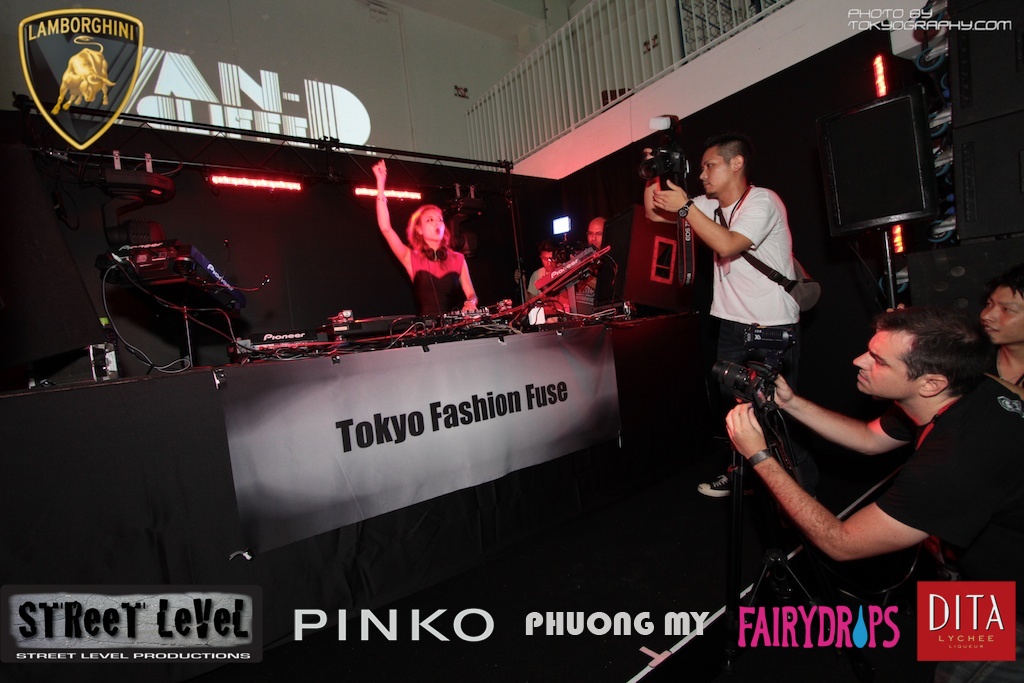The full-color indoor photograph captures an energetic scene at an automotive event. Dominating the stage, a woman wearing a sleeveless black dress with a pink bodice stands behind a DJ setup complete with turntables and an array of other audio equipment. She exudes confidence, raising one hand enthusiastically into the air while over-the-head earphones rest around her neck. The stage features a banner reading "Tokyo Fashion Fuse" and is positioned under a white-railing balcony with a black backdrop and some lighting highlights.

In both top corners, you find logos: the iconic gold Lamborghini emblem in the upper left and "photo by Tokiography.com" in the upper right. Surrounding the DJ, several photographers and paparazzi focus their lenses on her, capturing the moment. The bottom of the image displays an array of logos from event sponsors, including Street Level Productions, Pinko, Fyongmai, Fairy Drops, Dita, and Lychee. Additionally, a light above the DJ illuminates a wall sign reading "Van D Life," contributing to the vibrant atmosphere of the event.